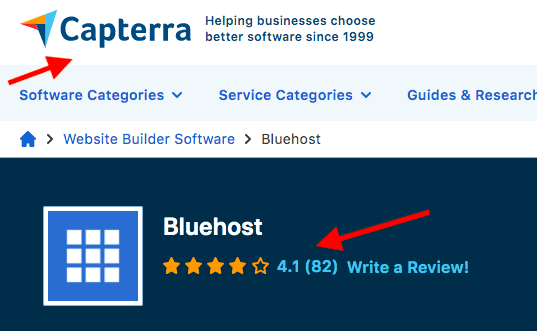This screenshot showcases the homepage of the CAPTERRA website, highlighted by its distinct logo positioned in the upper left corner. The logo features a color scheme of yellow, light blue, and dark blue. Immediately to the right of the logo, the tagline "Helping businesses choose better software since 1999" is prominently displayed. Under this tagline, three navigation sections are listed: software categories, service categories, guides, and research.

In the upper left corner of the screenshot, a red arrow has been placed beneath the word "CAPTERRA" to draw attention to it. Additionally, the primary focus of the webpage is not visible within the screenshot; instead, what takes up much of the view is an advertisement for Bluehost, a web hosting service. This advertisement is encapsulated in a large dark blue rectangle, with the word "Bluehost" displayed in white lettering.

Another red arrow points towards the reviews for Bluehost within this advertisement, indicating a rating of 4.1 out of 82 reviews, which translates to approximately a 4-star rating out of 5. The Bluehost logo consists of a large white outlined square with a light blue center, inside of which are several smaller white squares, forming a grid-like pattern.